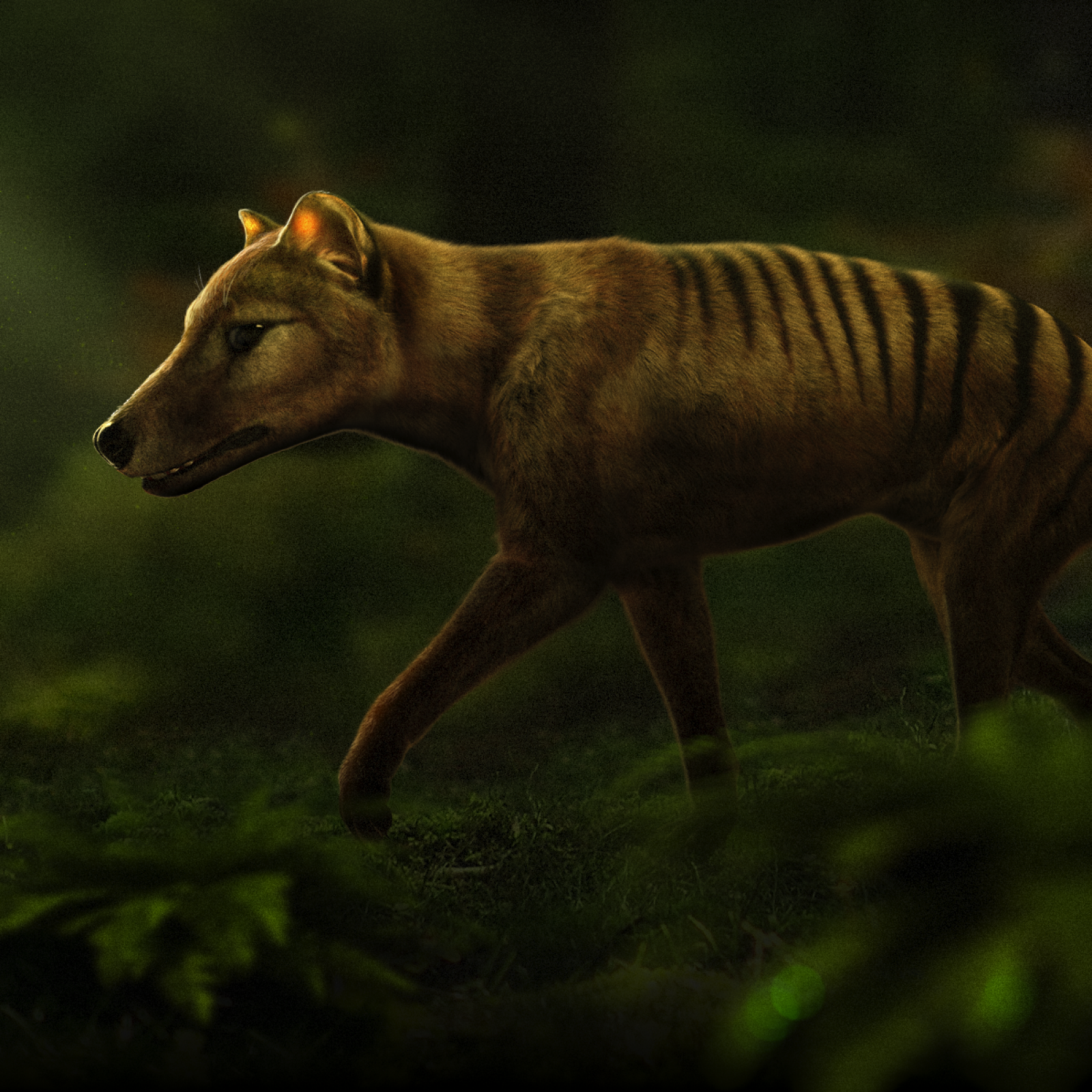The image features a digitally rendered animal, resembling a striped hyena, centrally positioned against a dark, green, jungle-like background. The creature exhibits a mix of traits from different animals: it has a long snout and a large black nose, reminiscent of a dog or hyena, and short, pointy ears. Its eyes are slightly larger and protrude backward. The animal's hindquarters are adorned with zebra-like black stripes, lending it a somewhat prehistoric appearance. This dog-like creature has a medium-sized body and appears to be moving from right to left, potentially on the hunt. The overall lighting is dim, with only the top portion of the animal subtly highlighted, adding to its mysterious presence. The background and foreground are filled with green vegetation, which is mostly out of focus, further emphasizing the central focus on this unique animal in its jungle setting.